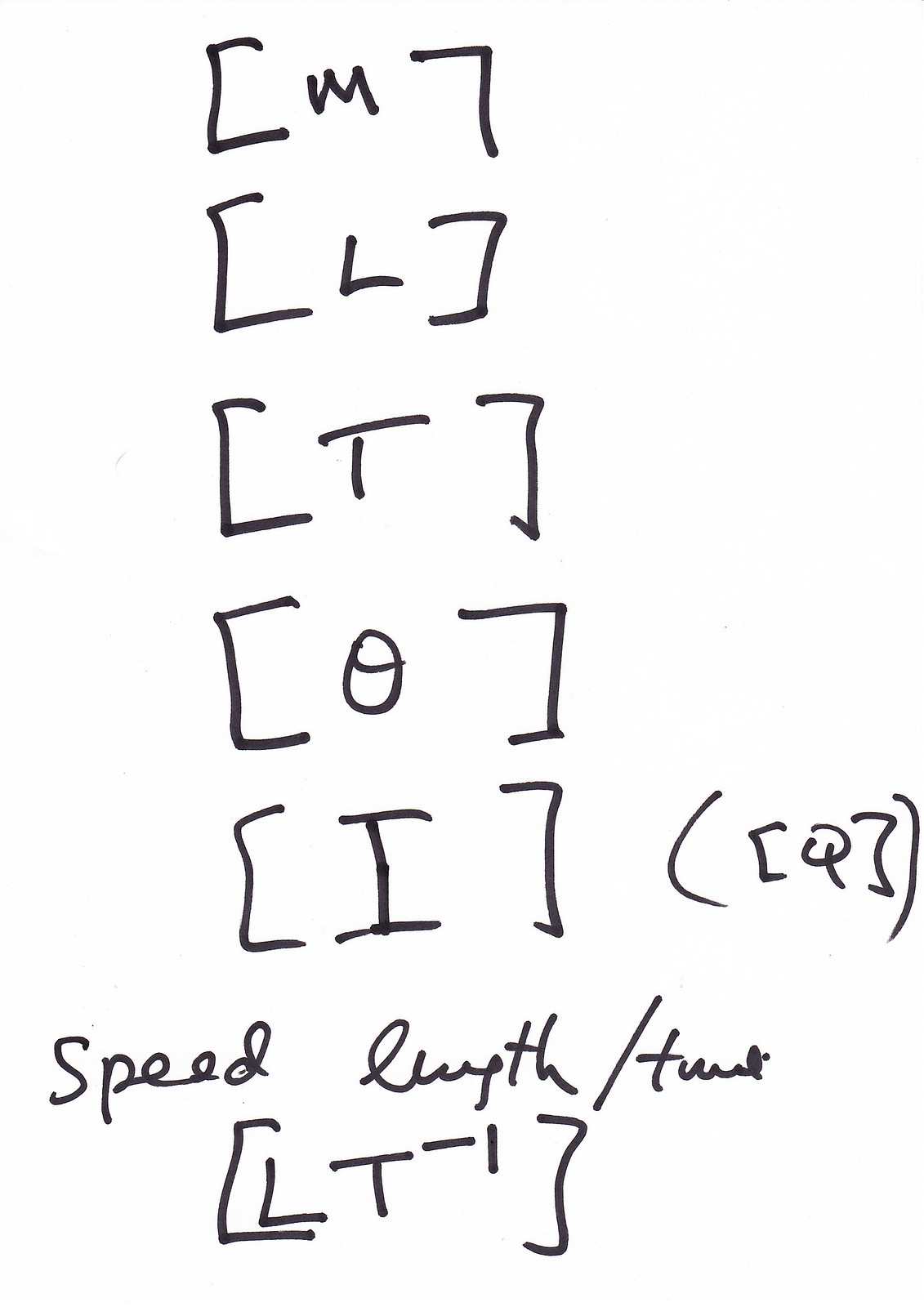The image depicts a digital note, likely created using a handwriting tool on a notepad app, featuring a crisp, white background. The handwriting appears to be in black ink, possibly mimicking the appearance of a Sharpie marker. The note includes the sequence of characters "M-L-T-O-I" enclosed in brackets, as well as individually bracketed letters, with a notable "Q" inside parentheses. Additionally, the text contains the words "speed," "length," and "over time," followed by "L-T-1" in brackets. The overall presentation suggests it might be a high-quality scan of handwritten material or a careful digital recreation, potentially related to a mathematical formula or notation.